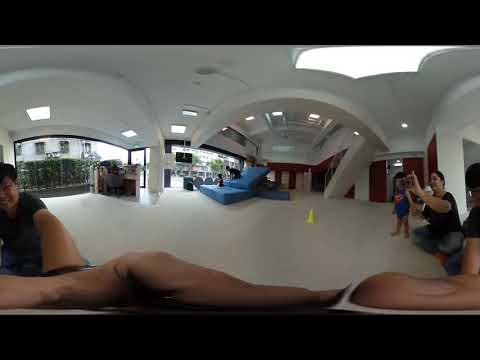The photograph captures the interior of a large, expansive white room, possibly a commercial space or hotel lobby, characterized by its open area, arched white ceiling, and curved white walls with recessed square lights. A panoramic shot reveals some distortion, highlighting an arched roof with sunroofs that indicate it is daytime. Central in the image is a large blue sofa surrounded by an open space with white floors and a small yellow cone. 

On the right side of the image, a woman wearing jeans and a black short-sleeved shirt is seen taking a photograph with her cellphone. Next to her is a young child, also in blue, possibly a toddler, though their face is not clearly visible. Additionally, a man, possibly Asian, wearing a black t-shirt and dark slacks is squatting and taking a selfie with another child at his side, also dressed in dark clothing. In the foreground, there appears to be a brown object, possibly the back of a sofa or seating area, while white stairways and doorways are visible on opposing sides of the room.